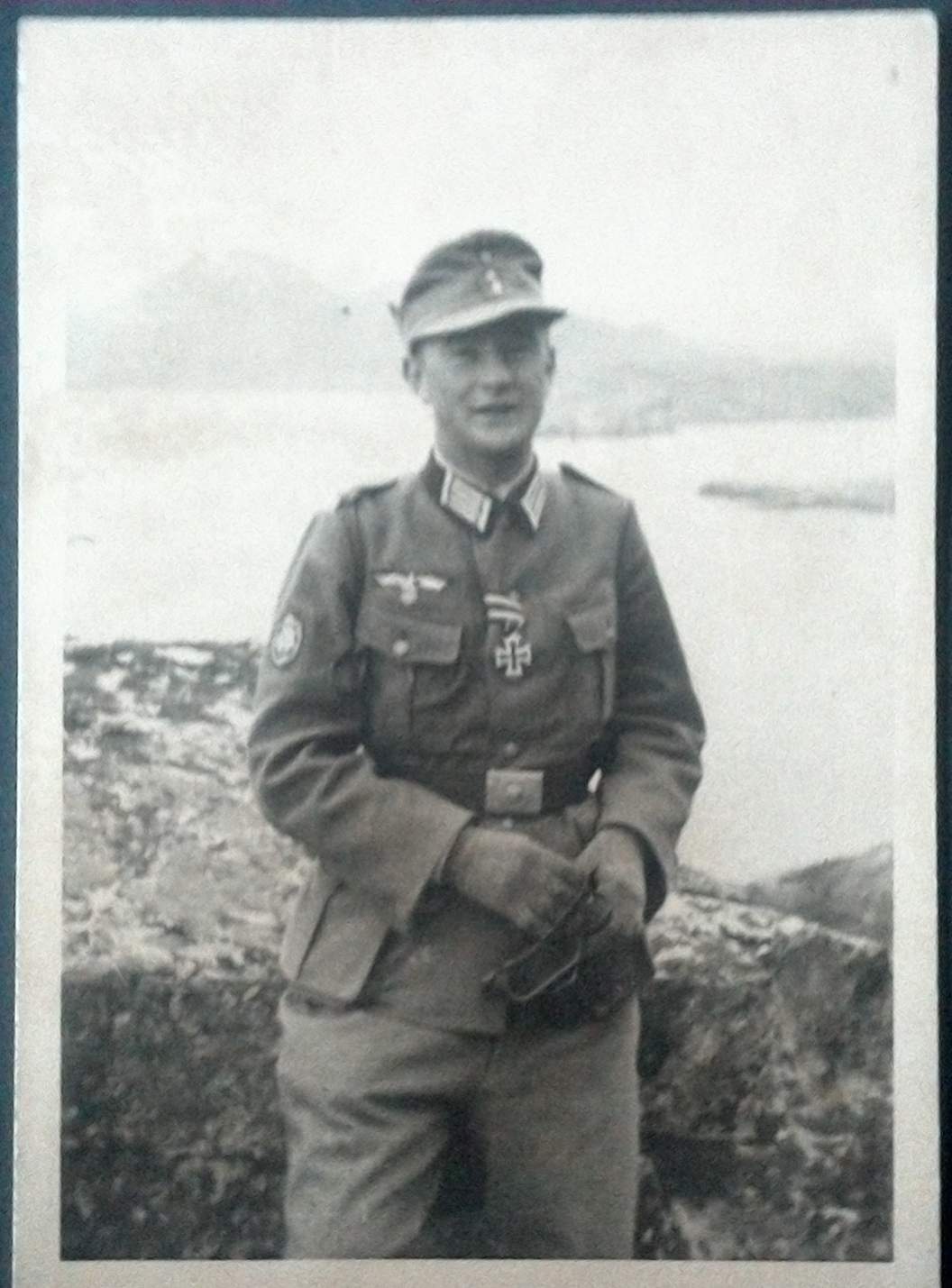This vintage black-and-white photograph, likely from the 1940s during World War II, features a German soldier in full military uniform. The scene is set with the soldier standing and leaning against a rock formation, with an out-of-focus body of water, possibly a lake or bay, in the background. The soldier is captured from head to about knee-length, facing the viewer directly. His uniform is adorned with several notable medals and insignia: a German knight's cross around his neck, a cross-shaped medal in the center of his chest, bars or special award-type insignia on his collar, a metallic emblem with an eagle above the right front pocket of his jacket, and another undecipherable emblem on his right arm. He also wears gloves and a classic military cap with a visor and an insignia on the front. In his crossed hands, he appears to be holding a small pouch or potentially a pair of goggles. The vintage photographic style emphasizes the historical and somber atmosphere of the era.